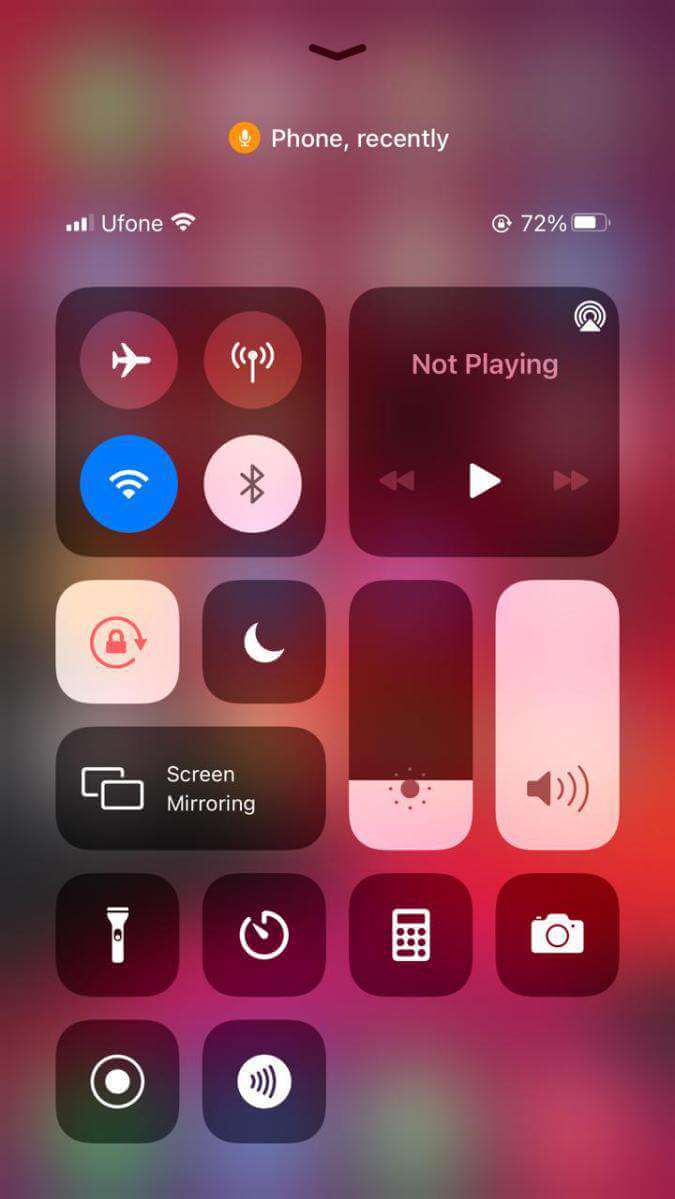Screenshot of an iPhone Control Center with various features. 

The background is blurred. At the top, there is an "orange microphone" icon next to the label "Phone." Below that, battery info is displayed with "iPhone, Wi-Fi, 72%."

In the main Control Center area: 
- A box with four circular icons: Airplane mode, Mobile Data, Wi-Fi, and Bluetooth.
- A music box labeled "Not Playing" with play, back, and forward controls.
- A screen lock icon.
- A "Do Not Disturb" moon icon.
- Screen Mirroring button.
- A flashlight button.
- A screen recording button.
- A clock icon, which likely represents the Timer.
- A speaker icon.
- A calculator icon.
- A camera icon.
- A brightness slider, currently set to a low level.
- An audio volume slider, currently set to full.

These are the main features visible in this Control Center screenshot.